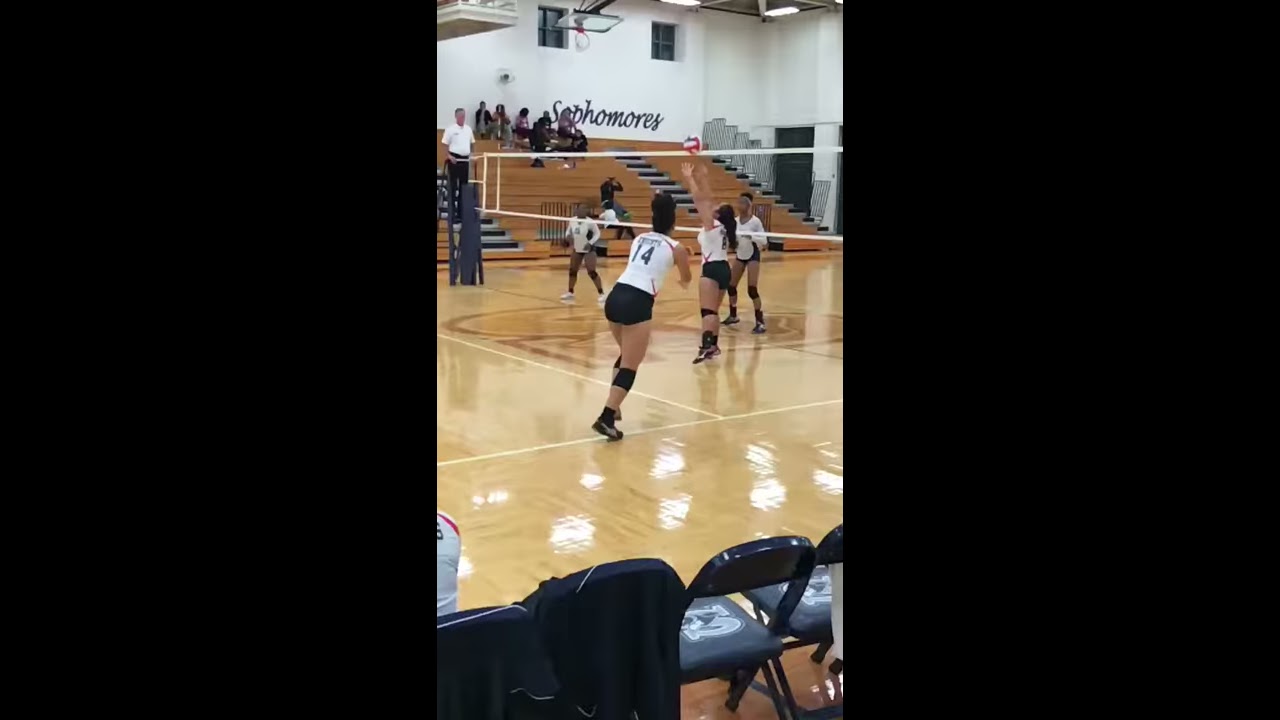In this detailed image of a high school girls' volleyball match taking place in a gymnasium with a wooden floor, the focal point is the action in the middle of the court where a player is setting the ball for number 14, who is poised to spike it at the net. Both teams are wearing white shirts with numbers and black shorts, which is unusual as teams typically have different colored jerseys. The volleyball itself is a mix of red, white, and blue. To the left, a referee is positioned in his stand, overseeing the game. The gym features wooden bleachers on the back wall, with a white wall above that includes black cursive wall art reading 'sophomores', likely indicating a section for sophomore spectators, although the few people seated there do not appear to be students. Near the ceiling, a basketball hoop is swung up out of the way. In the forefront, along the bottom of the image, there is a row of metal folding chairs marked with an 'S,' suggesting the home team's school name begins with this letter. The gym's environment, complete with low bench chairs and several fans, conveys the lively atmosphere as the game unfolds.